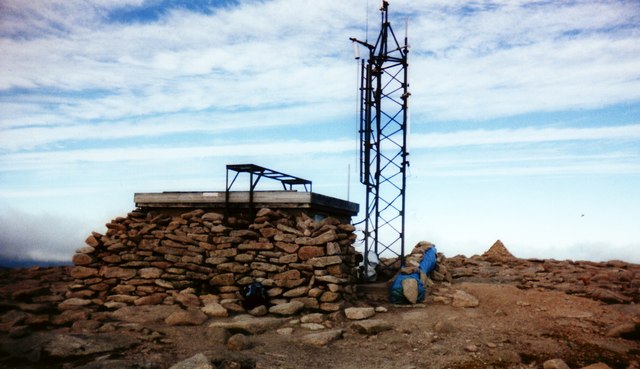The color photograph depicts a desolate landscape, likely a desert, with a prominent, horizontally oriented, deteriorating stone building situated in the foreground. The building, constructed from rough brown stones, appears to be crumbling, with a concrete roof topped by a horizontal metal structure resembling a ladder. Adjacent to the building on the right is a tall, black metal radio antenna, its base visible but the top extending out of frame. Emerging from the left of the building, wiring connects it to the antenna. Behind the building, a blue tarp is visible, possibly attached to the ground, while a solitary mountain looms in the background. The sky, occupying about 60-75% of the image, is mostly blue with streaky white cirrus clouds that thicken toward the horizon. The ground is a mix of brown earth, dirt, and scattered rocks and wood, enhancing the sense of isolation in this barren, natural setting.